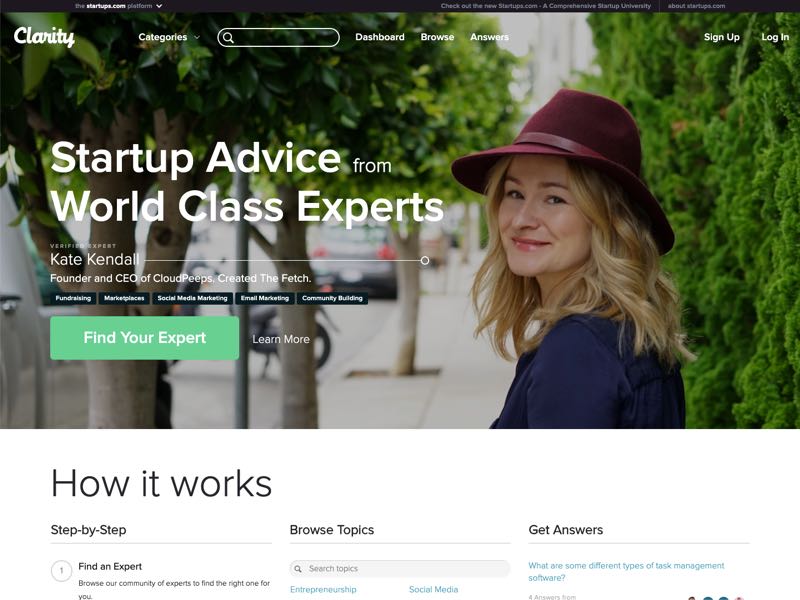This image showcases a webpage designed for providing clarity in various categories, with a search field positioned to the right. The top navigational links guide users to their dashboard, browsing options, answers, signup, and login sections. The page also features startup advice from world-class experts, prominently highlighting a smiling woman wearing a red hat, who is looking directly at the camera. In the background, lush green trees, parked cars, and a motorcycle add to the scene's vibrancy. The webpage outlines how the platform works, detailing steps such as finding an expert, browsing topics, and getting answers. It prominently lists task management software as a specific topic. Additionally, the page features a "Find Your Expert" section and a "Learn More" link, showcasing Kate Kendall, the founder and CEO of CloudCaps, who created a service called Fetch.